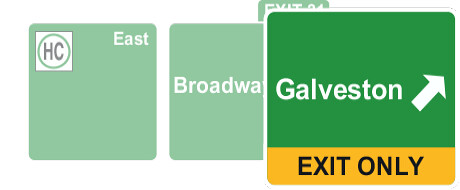This digitally-created image showcases a series of highway signs, predominantly rectangular and square in shape, with a primary focus on a clear and sharp sign on the right-hand side. The most prominent sign is rectangular and vividly displays the word "Galveston" in white lettering, accompanied by a bold white arrow angled upward from the lower left to the upper right. Below this is a yellow strip with the text "Exit Only" in black letters. Behind the Galveston sign, there are two slightly faded green signs with white lettering; one reads "Broadway" and the other, on the left, features a white square with a green circle enclosing the black letters "H" and "C," and the word "East" in white letters on the upper right-hand corner. In the distant background, just above the upper left corner of the Galveston sign, a faint sign indicates "Exit" followed by an indistinct number. The image contains no people and is characterized by its meticulous digital construction.